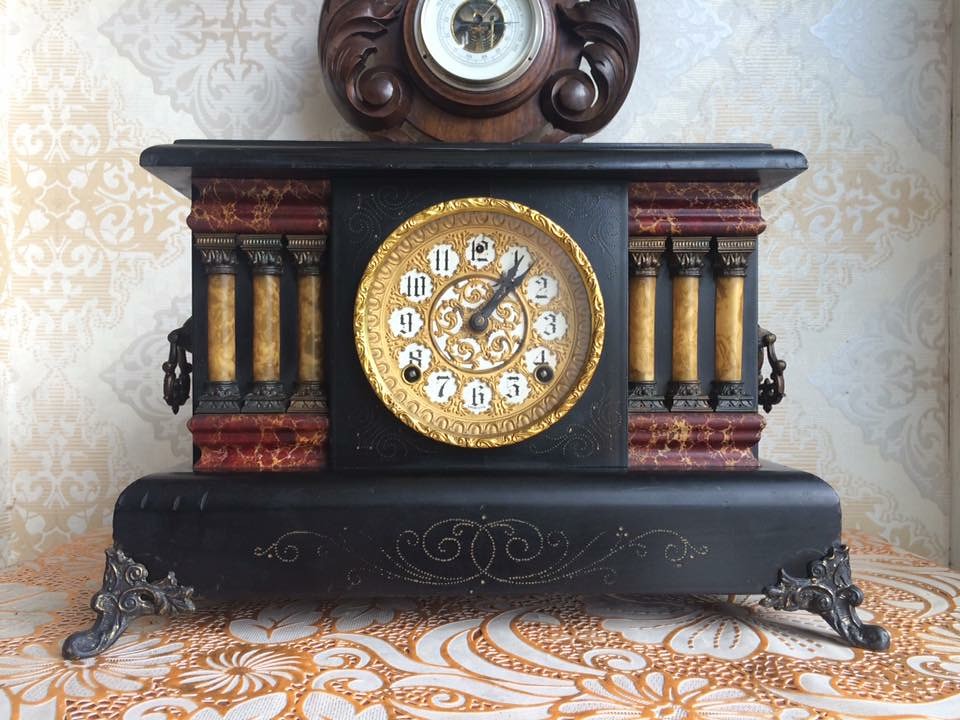The image depicts an antique mantel clock positioned on a tablecloth. The clock's wide base, which appears to be made of wood, is painted black. It features an intricate white etching design along the bottom, though part of this design is worn off, hinting at the clock's age. Elaborately crafted metal feet enhance the corners of the base.

The clock is set on a tablecloth adorned with a brown background, highlighted with swirls of white and flowers detailed in white with brown outlines. The base of the clock showcases three mustard-colored columns on each side, resembling marble pillars. These pillars are supported by maroon sections with brown lines woven throughout, enhancing the antique aesthetic. 

On both ends of the clock, metal rings hang down, adding to its ornate design. The clock's top surface is a black platform. Resting atop it is a round, sculpted piece of wood with swirls surrounding a solid brown ring. The center of this wooden structure features a transparent round window through which the intricate mechanics of the clock are visible, adding a fascinating element to its antique charm.